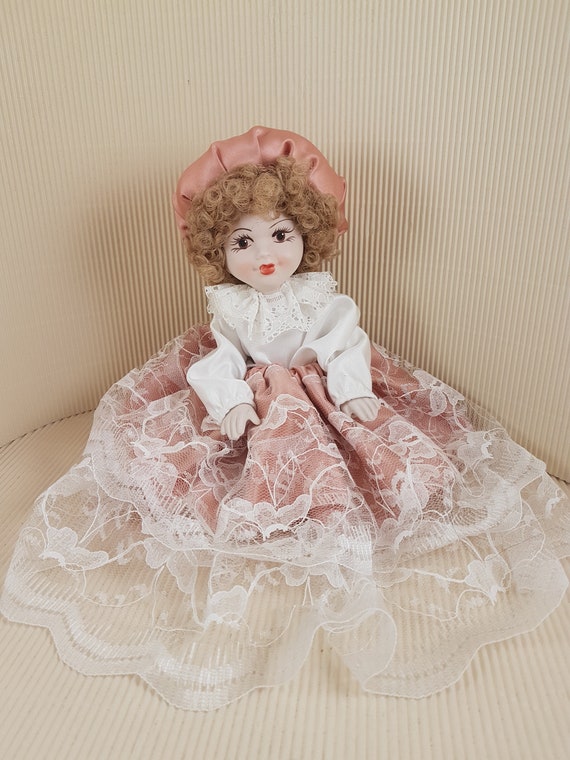The image showcases an exquisite porcelain doll with intricately painted features. She has vibrant red lips and deep dark brown eyes. Her hair is composed of synthetic curls in shades of blonde and brown, beneath a pink hat that sits elegantly at the back of her head. The doll is dressed in a white satin long-sleeve blouse adorned with a large lacy collar, paired with a pink dress featuring floral patterns and an overlay of delicate white lace. Positioned in the corner of what appears to be a display box or perhaps the corner of a room, the background is uniformly beige, as is the ribbed couch or floor on which she sits. The overall setting suggests it could be part of a storefront advertisement or a promotional display for the doll.